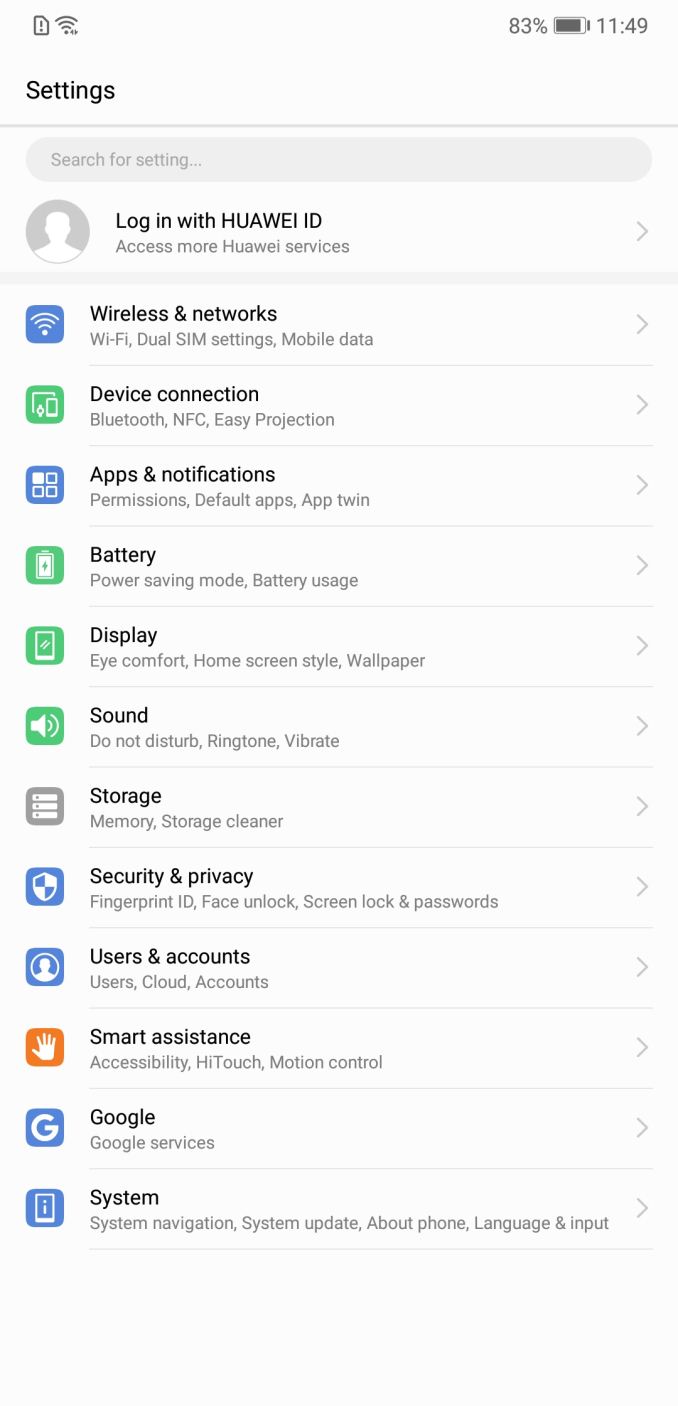Displayed is a screenshot of the settings section on a mobile device. The background of the entire image is white, providing a clean canvas for the various settings options. At the top left corner, the word "Settings" is prominently displayed in bold text. Directly beneath this, there is a search bar where users can type in keywords to find specific settings. Below the search bar, there is a section for the user’s Huawei ID, encouraging the user to log in with the message, "Access more with Huawei services."

Following this are categorized settings options listed in a vertical sequence:

1. **Wireless & Networks** 
2. **Device Connection**
3. **Apps & Notifications**
4. **Battery**
5. **Display**
6. **Sound**
7. **Storage**
8. **Security & Privacy**
9. **Users & Accounts**
10. **Smart Assistance**
11. **Google**
12. **System**

Each category is clearly labeled, making it easy for users to navigate and manage their device settings efficiently.